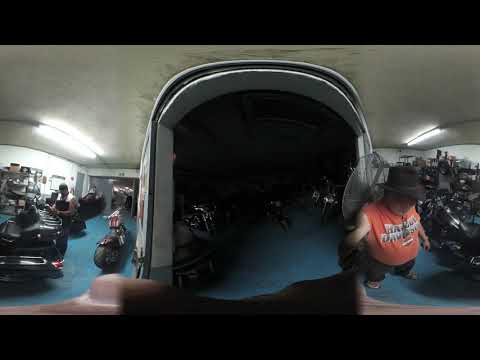The image depicts a distorted, composite scene presumably taken with VR that combines three separate photos merged together, bordered by black rectangles at the top and bottom. Inside a large, dimly-lit room with a blue carpet, there are numerous motorcycles parked and not in use. On the left side, partially visible under fluorescent ceiling lights and white ceiling tiles, stands a heavyset Caucasian man wearing a black hat and jeans, seeming to work on the motorcycles. The center of the image features a white arched entrance leading into a darker area filled with more motorcycles. On the right side, another Caucasian man appears unusually small, possibly due to image warping. He wears a distinctive sleeveless orange Harley Davidson shirt, a brown bowler or cowboy hat, black pants, and possibly flip flops. The room's interior displays a somewhat chaotic layout due to the visual distortions, contributing to a sense of disorientation.